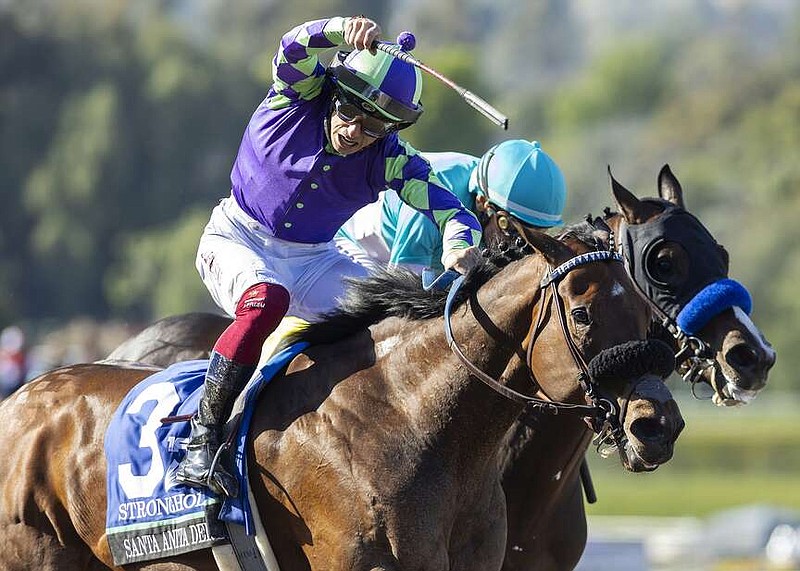The image depicts a thrilling horse race featuring two brown horses, each ridden by a jockey. Both horses wear eye patches to prevent them from getting spooked or distracted. The horse on the left is a lighter shade of brown and sports a blue cloth with the number three visible. The jockey on the left is dressed in a vibrant purple and yellow outfit, complete with a checked jersey on the sleeves, a matching helmet, sunglasses, white shorts, red socks, and black boots. His right hand grips a whip poised in the air. The jockey on the right is clad in light blue and white, including a light blue hat. Both horses have black manes and wear black masks, along with thick straps around their nose area. The background is a blur of green, filled with tall trees and a green grass field, with some spectators discernible in the lower left corner. This action shot captures the intensity and excitement of the race, with the horses neck and neck.